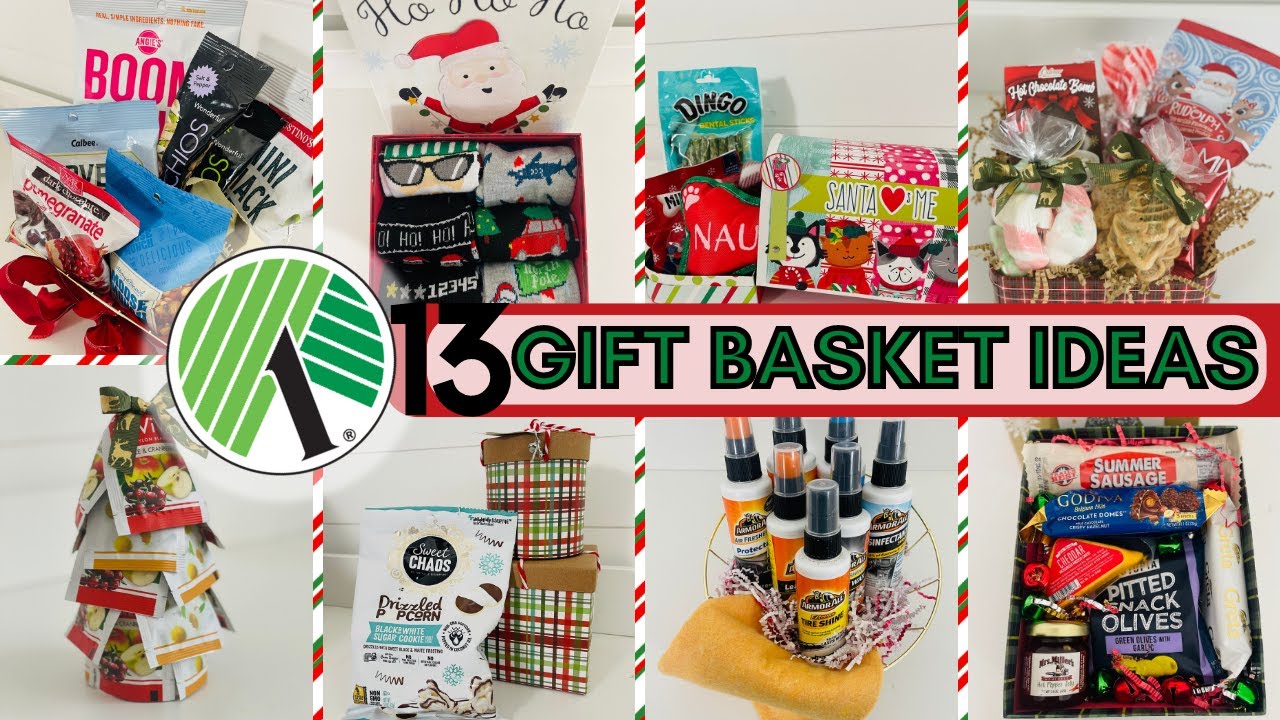This colorful Dollar Tree advertisement showcases 13 creative gift basket ideas, perfect for the holiday season. The image is divided into eight smaller sections, each highlighting a different theme. In the upper left, an assortment of snacks is displayed, followed by festive Christmas-themed socks, assorted candies, and a mix of toiletry and candy items on the right. Centrally positioned is the Dollar Tree logo, emphasizing the holiday spirit with vibrant colors. The bottom row includes a unique Christmas tree made from packet items, gift boxes with drizzled popcorn, a basket filled with various bottles, and a charcuterie-themed basket featuring pitted olives, summer sausage, and other gourmet snacks. The diverse selection illustrates multiple thoughtful and budget-friendly gift options, making holiday shopping easy and enjoyable.